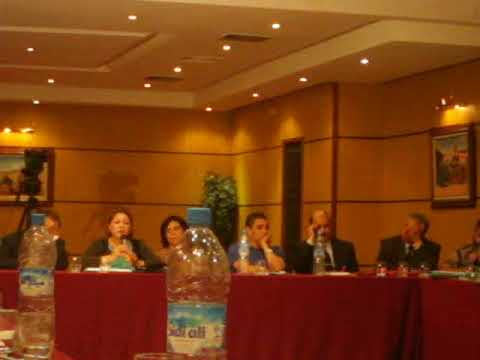The image depicts an indoor conference or possibly a press event, set within a conference room or hotel banquet area. The central focus is a panel of seven individuals seated at a long table draped with a red tablecloth, engaged in a serious discussion. All panelists are provided with bottled water, some of which are clearly visible at the bottom of the image. One woman on the panel is prominently featured holding a microphone, suggesting she is currently speaking. The room's décor includes orange and red walls adorned with artwork, and overhead, recessed lighting emits a yellow-gold hue. The setting conveys a formal atmosphere, with participants deeply engrossed in the conversation, some taking notes and others contemplating the issue at hand.